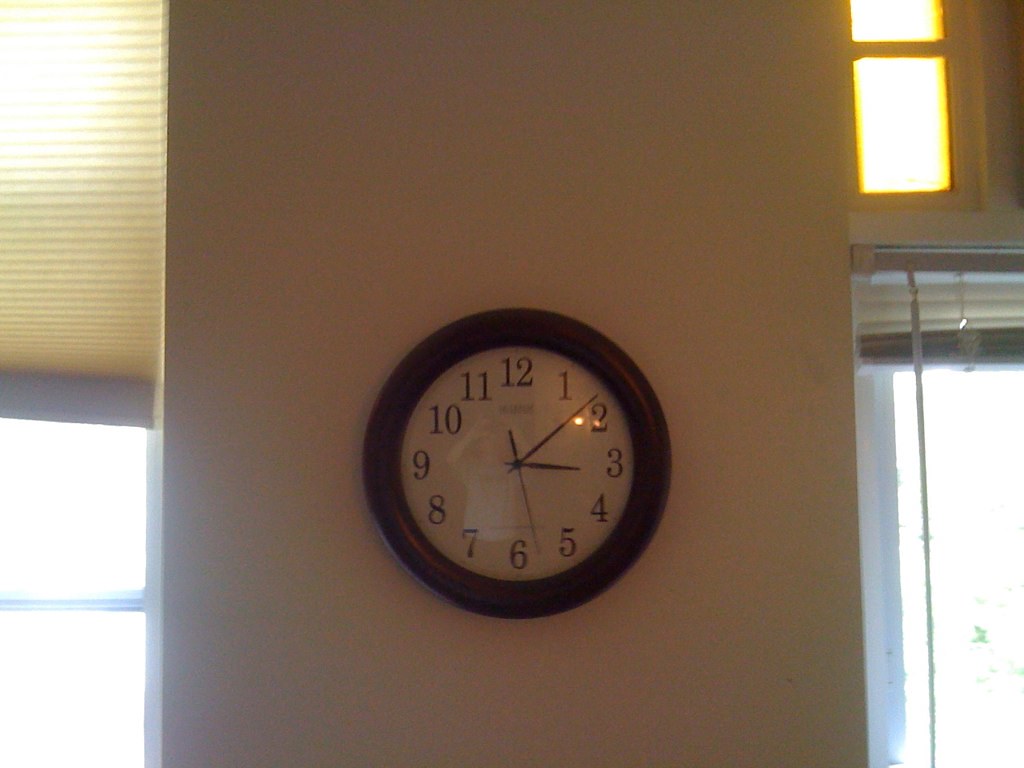This photograph captures a round clock prominently displayed in the center of a beige wall, which appears to be situated between two windows. The wall looks somewhat temporary or partition-like. The clock features a dark wooden trim with a dome-shaped glass cover, and a white face displaying traditional black numbers from 1 to 12. The thin, spindly black hour, minute, and second hands indicate the time as approximately eight minutes past three, with roughly 28 seconds. To the left of the clock, light streams in through a window partially covered by a half-drawn blind. On the right side, another window is fully exposed, with an additional small vertical window with a divider positioned above it. A long pole for adjusting the blind hangs to the right of the clock. Overall, the photograph provides a detailed depiction of the clock and its surrounding elements, emphasizing the interplay of light and structure within the space.